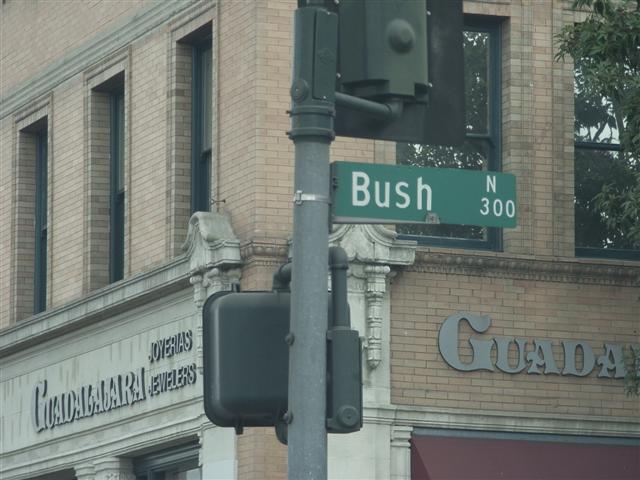This photograph captures a bustling street corner dominated by a metal street pole featuring a green street sign with white lettering reading "Bush." To the right of the street name, the sign displays an 'N' and '300' in white. The street pole stands in front of a brick building, constructed from light pine-colored beige bricks, identifying the corner of the edifice. On the left side of this corner, the building boasts a cement facade bearing the sign "Guadalajara Jewelry." The right side continues in the same brick texture, with the shop's signage mounted directly against the brickwork. Atop the pole, the backs of a traffic light and pedestrian signal subtly peek into view. A tree's branches emerge into the top right corner of the frame, adding a touch of greenery, while a vibrant red awning beneath the shop name draws attention in the bottom right corner, hinting at the lively atmosphere of the urban setting.